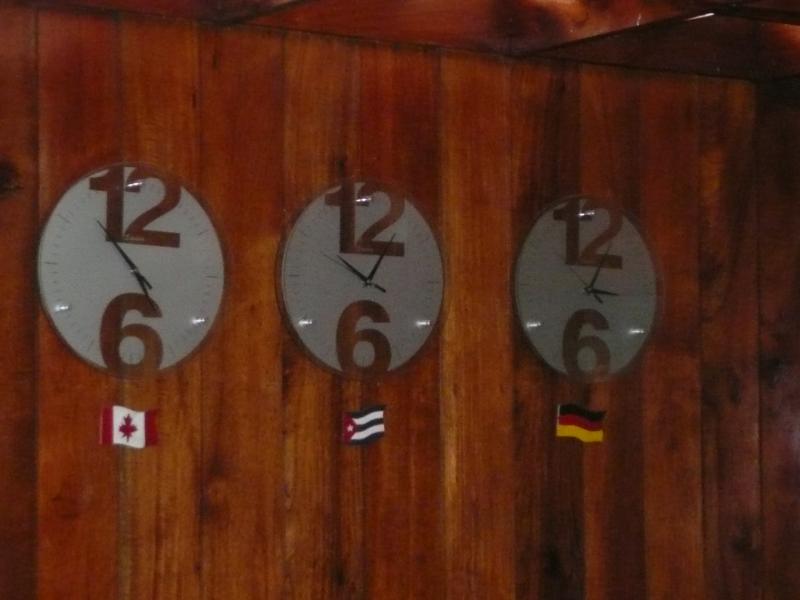This color photograph, taken indoors in landscape orientation, features a prominent wooden paneled wall that serves as the backdrop. The wood has a cherry oak finish with darker areas, almost approaching black, highlighting the natural knots and vertically running grain of the panels. Mounted on the wall are three identical clocks, each set to different time zones and aligned in a row. The clocks all have silver faces with oversized, transparent numbers 12 and 6, allowing the wood paneling to be visible through them. Each clock face includes hour, minute, and second hands, all positioned differently. Below each clock, enamel pin badges represent various countries: the left one displays the Canadian flag with its iconic red maple leaf, the middle has the North Korean flag featuring a sidewise red triangle and distinctive horizontal navy and white stripes, and the right one showcases the German flag with horizontal stripes of black, red, and yellow.